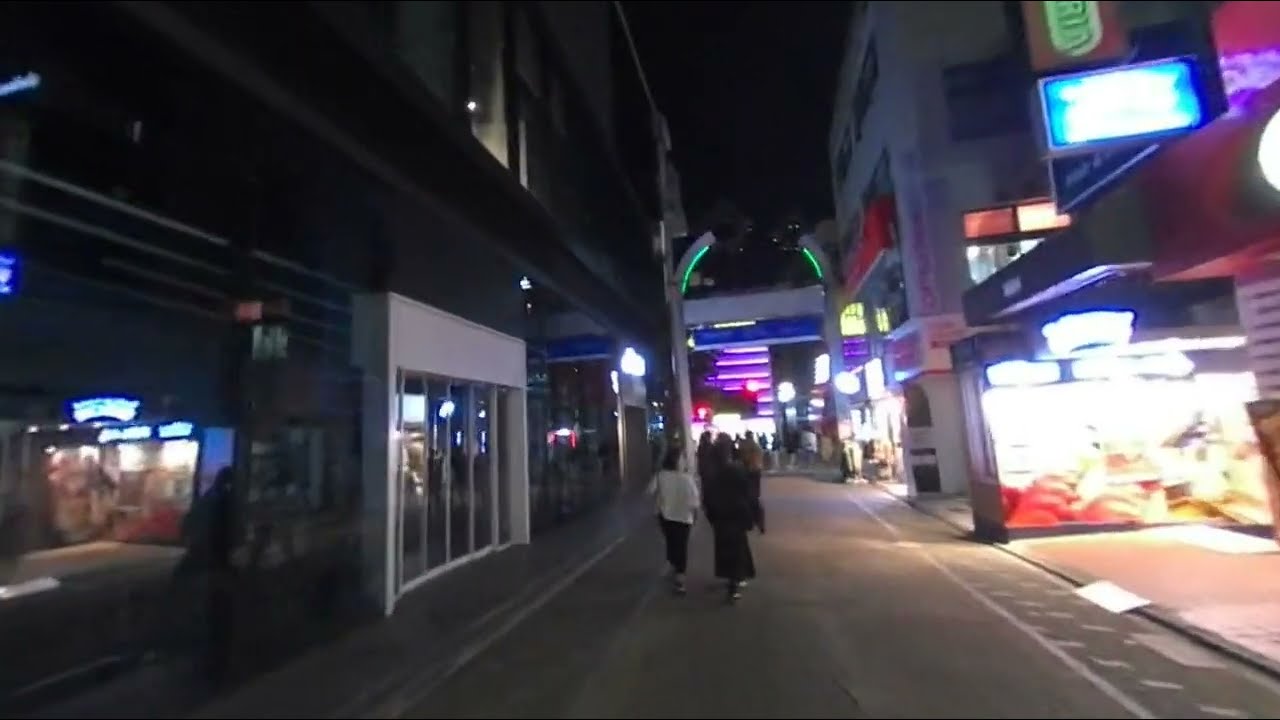This image captures a night scene on a pedestrian city street lined with commercial buildings on both sides. The left building is a three-story structure with numerous windows, while the right building features extensive lighting and advertising signs, particularly on its first and second floors, making the details difficult to discern. The street, devoid of vehicular traffic, is partially illuminated by green-tinged street lights and the glow from the buildings, which are predominantly black and white with blue trim and details. Two people are prominently visible from behind, walking side by side down the middle of the street; the person on the left, likely a woman, is dressed in a white top and black pants, carrying a purse over her shoulder, while the person on the right, possibly also a woman, wears a black dress or jacket. The scene suggests light foot traffic typical of a busy area during the day that has quieted down at night. Though other people are present further down the street, they appear indistinct and out of focus. A fast-food stall can be seen on the right side, adding to the commercial atmosphere of the area. The overall image may seem blurry, akin to a still from a video, giving a dynamic, in-the-moment feel.